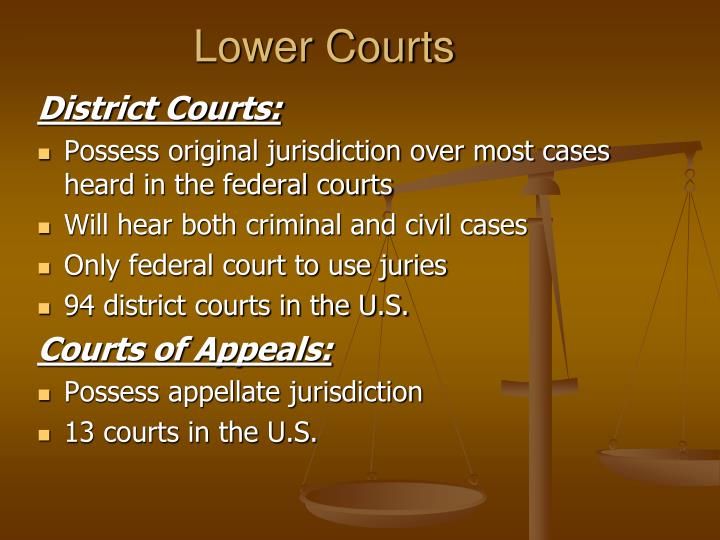The image appears to be a slide with an educational or informational purpose, likely from a PowerPoint presentation or learning aid, featuring a dark gold to yellow gold gradient background. In the lower right, there's a faint image of the scales of justice, adding a thematic visual element. The slide is titled "Lower Courts" in pale yellow, centrally located at the top. On the left side, underlined headings in light beige read "District Courts" and "Courts of Appeals."

Under "District Courts," there are four bullet points in white:
- Possess original jurisdiction over most cases heard in the federal courts.
- Will hear both criminal and civil cases.
- Only federal court to use juries.
- Ninety-four district courts in the U.S.

Under "Courts of Appeals," two bullet points read:
- Possess appellate jurisdiction.
- Thirteen courts in the U.S.